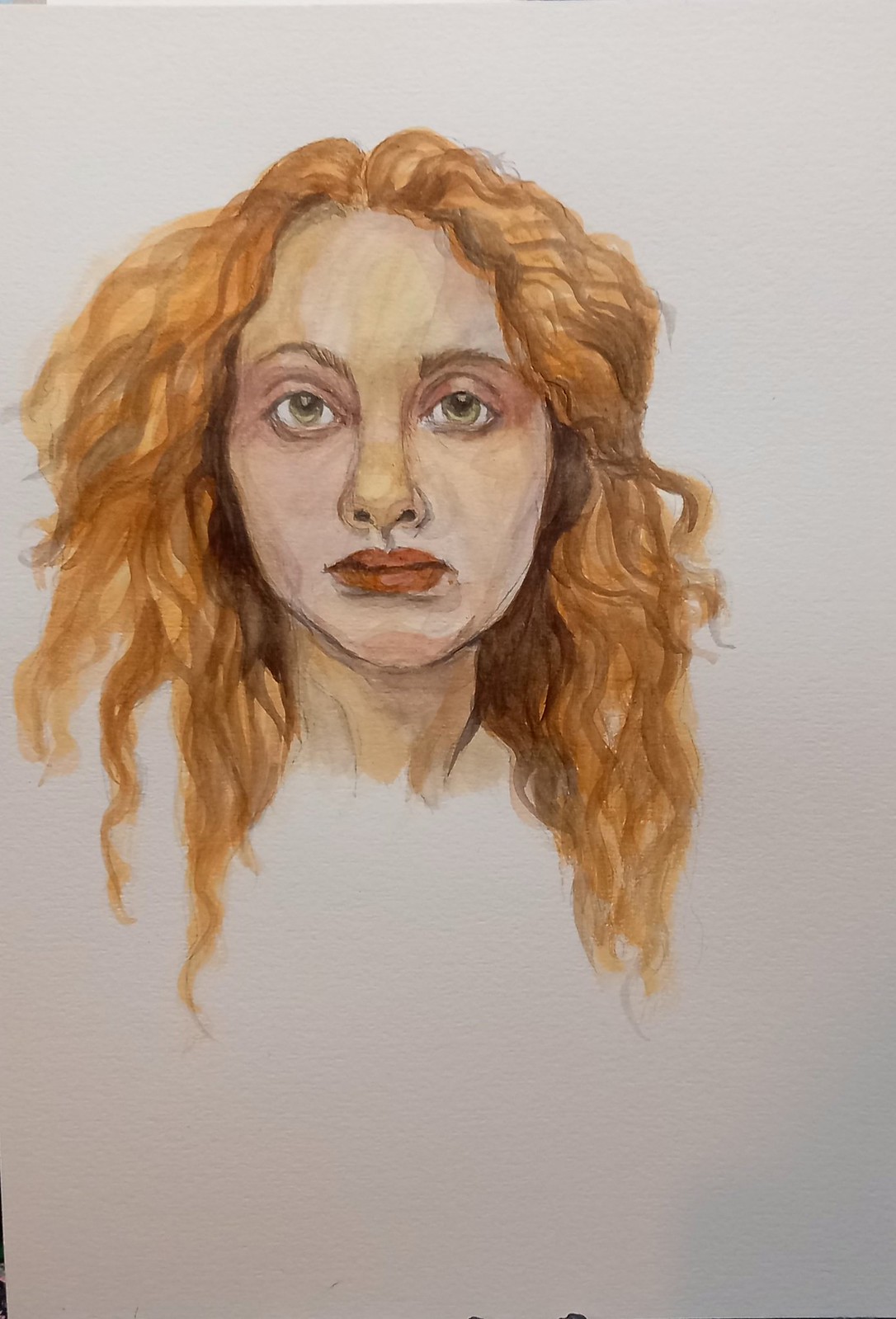The image is a handmade drawing of a white woman with pale skin and faint shading on her face. She features captivating green eyes with finely detailed irises and thin eyebrows. She has full red lips and shoulder-length, wavy red hair with lighter highlights, falling across both shoulders in long, layered strands. The composition reveals her slightly off-center, positioned toward the top left of a white sheet of paper, which seamlessly blends into a subtle gray background. Her expression is pensive, gazing into the distance with one eye slightly more open than the other, giving her a somewhat melancholic appearance. The artwork, done in color resembling a mix of colored pencil and watercolor, displays her from the neck up, with her neck depicted clearly while the rest of her body dissipates into the white background, leaving a semi-professional yet unfinished impression.